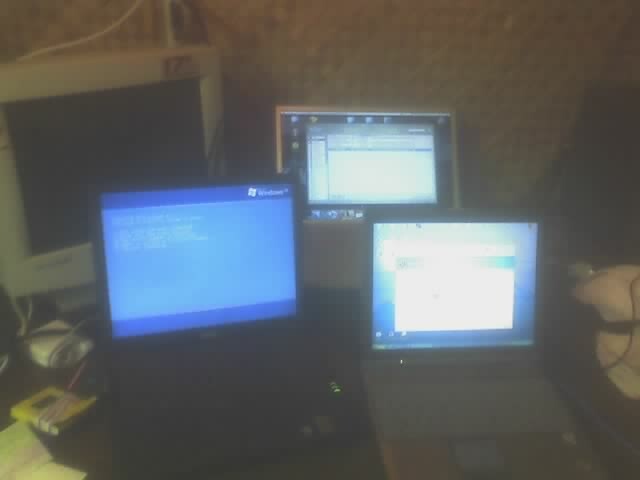The image is a blurry, low-quality photograph depicting a collection of four old computers on a desk. The setup includes one desktop computer in the back left, which is a large, boxy CRT monitor in a grayish color and is turned off. In front of it sits a black laptop displaying a Windows boot-up screen. To the right of this black laptop, slightly elevated, is a gray laptop with a window open on the screen, possibly displaying the file system. Below this gray laptop, another similar gray laptop has an open window with a blue screen and a white screen inside of it, though the details are unclear due to the blurriness. All devices are resting on a flat surface or table, with a dark or black color. The background of the image appears to be indistinct and a brownish color, adding to the vintage feel of the setup.